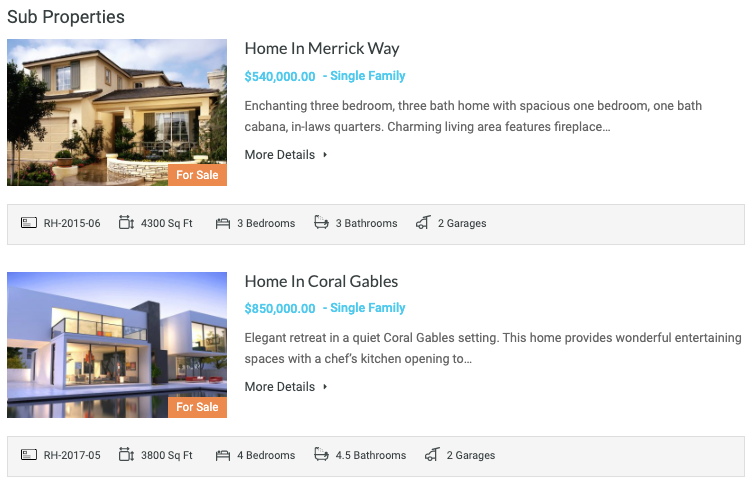**Website Screenshot of Property Listings**

The screenshot appears to be from a realtor's website, featuring "Sub Properties" in black font at the upper left-hand corner. Below the header is an image of a stone-clad house with a flat façade. The house includes a garage facing the camera on the left side and a picture window on the right. It has a brownish roof and a leafy tree partially visible on the left side of the image. At the bottom right corner of the picture, there's a "For Sale" sign, indicating that the house is available on Merrick Way for $540,000. This single-family home listing is accompanied by detailed descriptions such as square footage, the number of bedrooms, bathrooms, and garage spaces.

To the right of the Merrick Way listing, another property is showcased. This is a single-family home located in Coral Gables, priced at $850,000. Similar to the first listing, this property includes specifics about the square footage, bedrooms, bathrooms, and garage capacities.